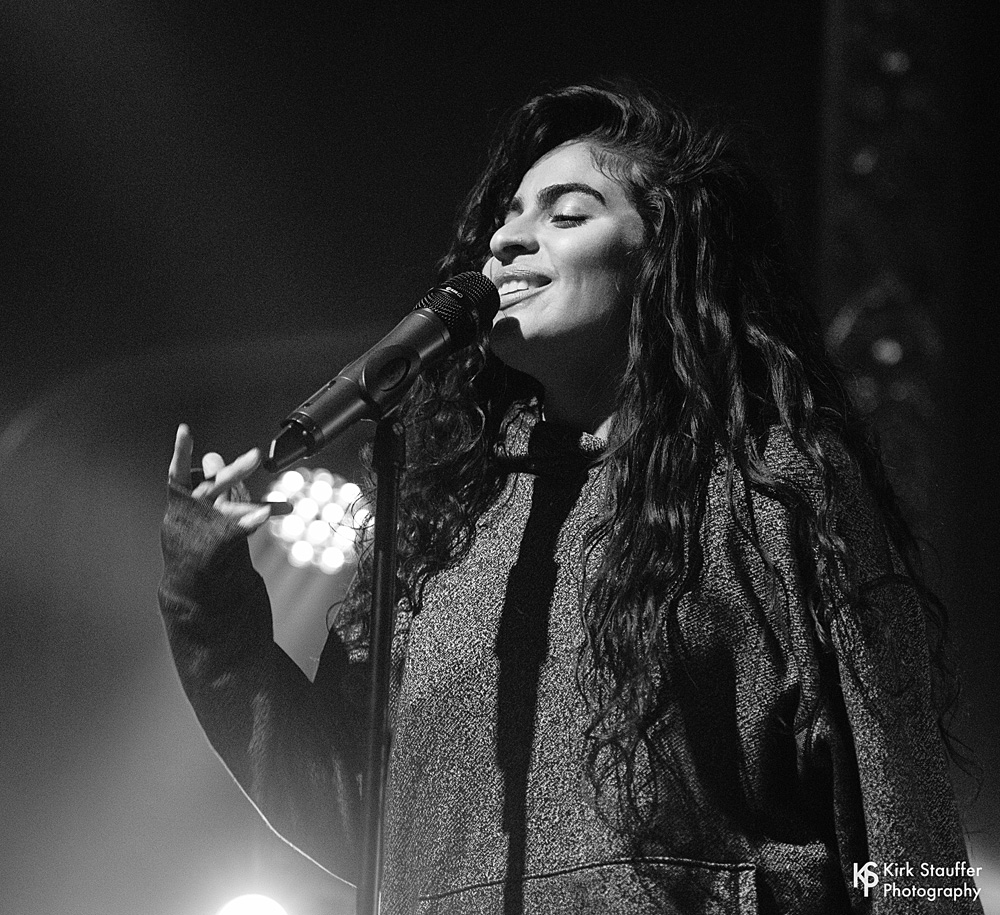This black and white photograph captures an evocative moment of a woman, possibly of Indian or East Asian descent, engaged in a vocal performance. She stands confidently behind a prominent, floor-standing microphone, with a subtle smile playing on her lips, revealing her upper teeth. Her eyes are closed, suggesting she is deeply immersed in her music. Her long, wavy hair cascades down to her waist, adding to the ethereal atmosphere of the image. She is dressed in a dark, dappled long-sleeved top that contrasts with the vivid lighting on her face and upper body. Interestingly, there's a digitally inserted, starkly white hand beside her own, indicating some form of photo manipulation. The microphone and its stand cast a distinct shadow on her chest, adding depth to the composition. The photograph is branded with "Kurt Stauffer Photography" in the bottom right corner, accompanying a stylized "K-S-P" logo.